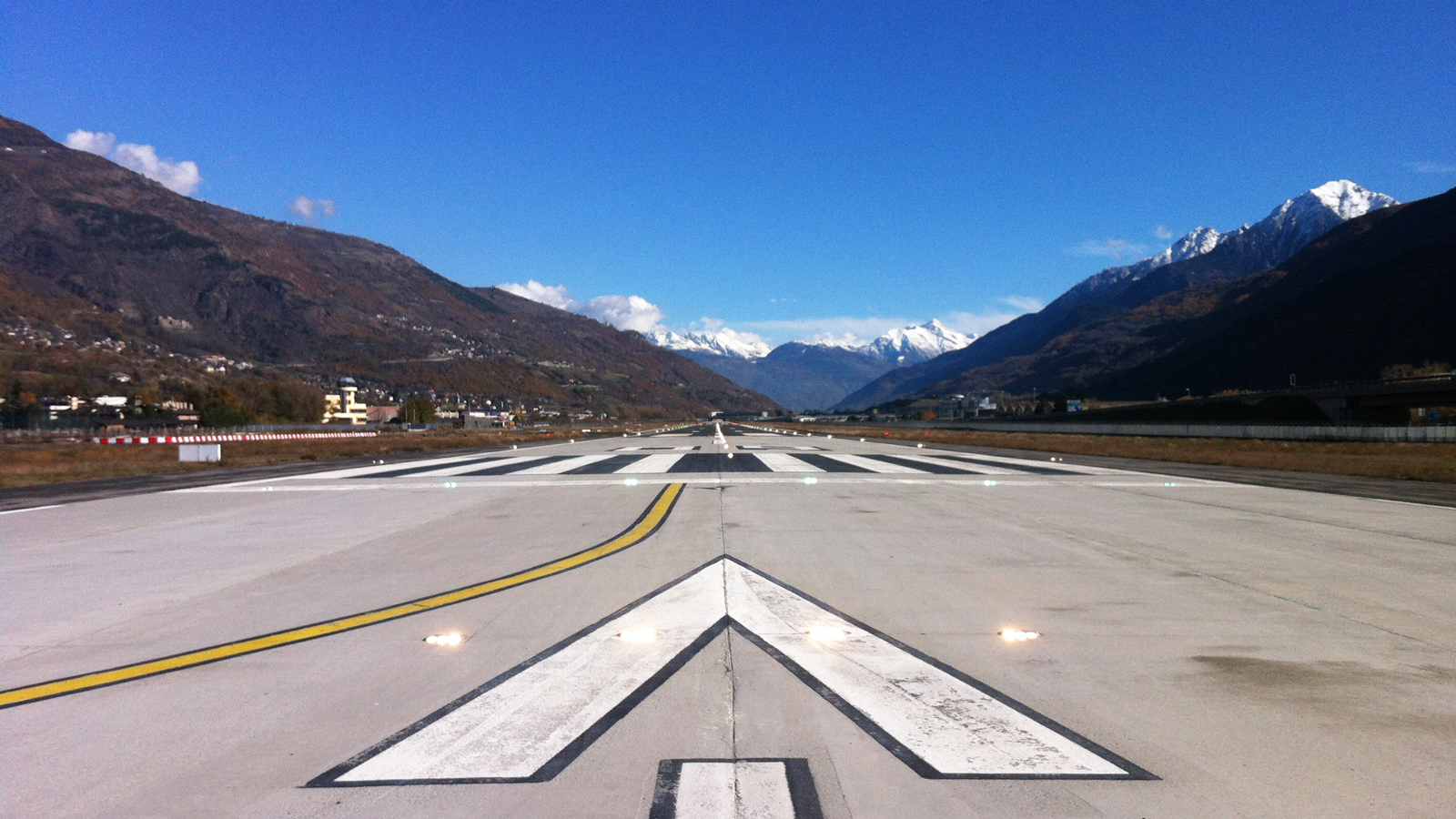The image presents a vibrant, daytime scene of an airport runway set amidst towering, snow-capped mountains under a deep blue sky adorned with scattered white clouds. The concrete runway, extending away from the viewer, is marked with a large arrow pointing forward, alongside an array of white and black cross stripes indicating the points for takeoff and landing. A curved yellow taxi line arcs onto the runway, guiding aircraft to their starting positions. Lit landing lights line both sides of the runway, contributing to the detailed infrastructure. To the left, the scene includes grassy areas, brown hills, and a section of airport infrastructure featuring a possible terminal, a control tower, and other scattered buildings, all nestled in the mountainous region. Similarly, the right side of the runway displays hilly terrains with a few nondescript airport buildings. The mountains frame the runway, rising dark green-brown in shadow, with further snow-capped peaks visible in the distance, enhancing the landscape's dramatic natural beauty.